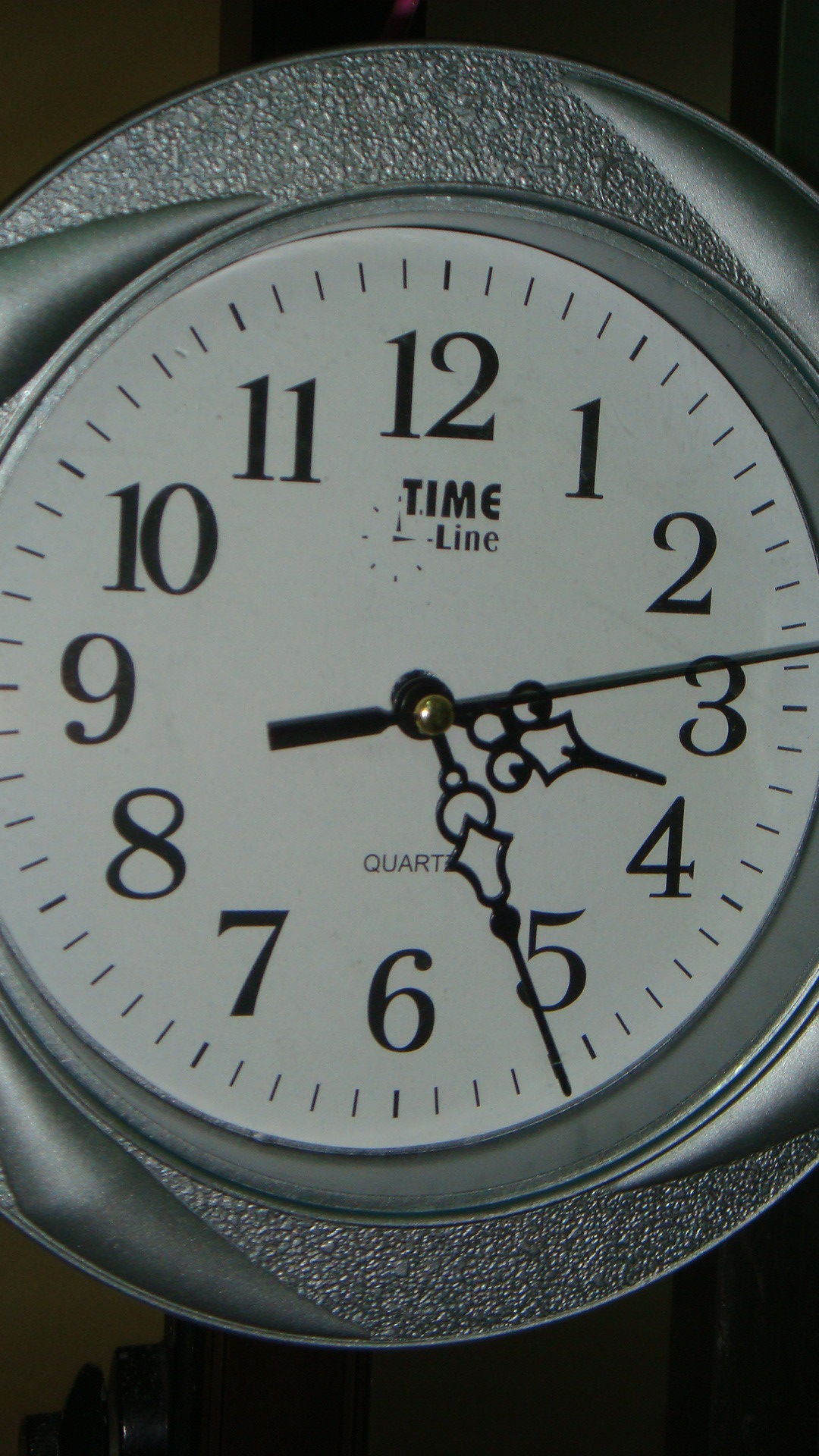The photograph captures a narrow view of a wall-mounted clock against a brown backdrop. The clock features a white face with large, black numbers from 1 to 12, accompanied by smaller black hash marks indicating the minutes. The hands of the clock, including the ornate second hand, are also black, standing out clearly against the white background. 

The clock's border is a combination of textured and smooth silver patterns, giving it a slightly antique or vintage appearance. This border includes a swirling design with raised, smooth sections that add depth and character. The outer trim of the clock has a gunmetal gray finish, further emphasizing its classic look.

Notable details include the text "Timeline" prominently displayed under the number 12 and the word "Quartz" beneath the center of the hands, both written in black. The overall design, with its intricate, textured border and distinct font, suggests a blend of modern and retro aesthetics, reminiscent of styles from the 1990s to the early 2000s.